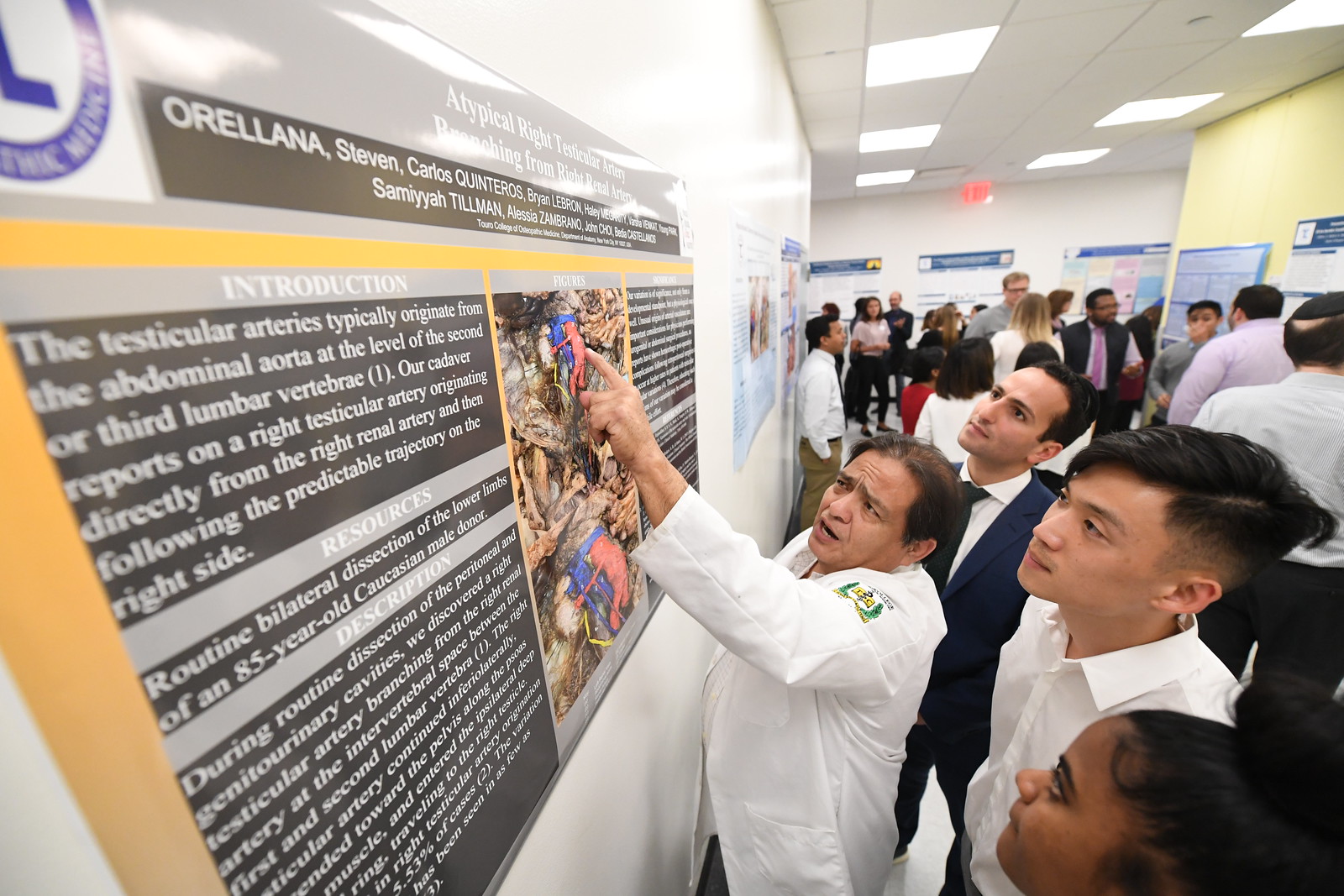This detailed photograph, taken in landscape orientation, depicts a bustling hallway inside a medical or healthcare conference facility, illuminated by fluorescent ceiling lights. In the foreground stands an Asian doctor wearing a white lab coat with a green insignia on the left shoulder, pointing at a large informational poster on the wall. His focused expression and pointed gesture towards the image of the human body's testicular arteries suggest he is explaining something crucial to a small group of attentive people. These individuals, consisting of another Asian man, a white person, and a black woman, are varying in dress from white medical coats to more formal dark suits, likely indicating a mix of medical professionals and conference attendees. 

Behind the main group, the hallway teems with activity. Around 20 to 30 people, of diverse backgrounds, some dressed casually and others formally, are engaged in various conversations or viewing other posters along the walls. There is a notable individual in the background wearing a yarmulke. 

The informational poster prominently features the name "Orellana Steven Carlos" at the top, followed by a heading labeled "Introduction." The text, in white against a brown background, provides detailed anatomical information about the testicular arteries originating from the abdominal aorta at the level of the second or third lumbar vertebra. A blue circle on a white background with an 'L' in the center, likely representing the conference's logo, is partially visible at the upper left corner of the poster. Additional posters and calendars are scattered on the walls throughout the hallway, enhancing the informative and scholarly atmosphere of the facility.